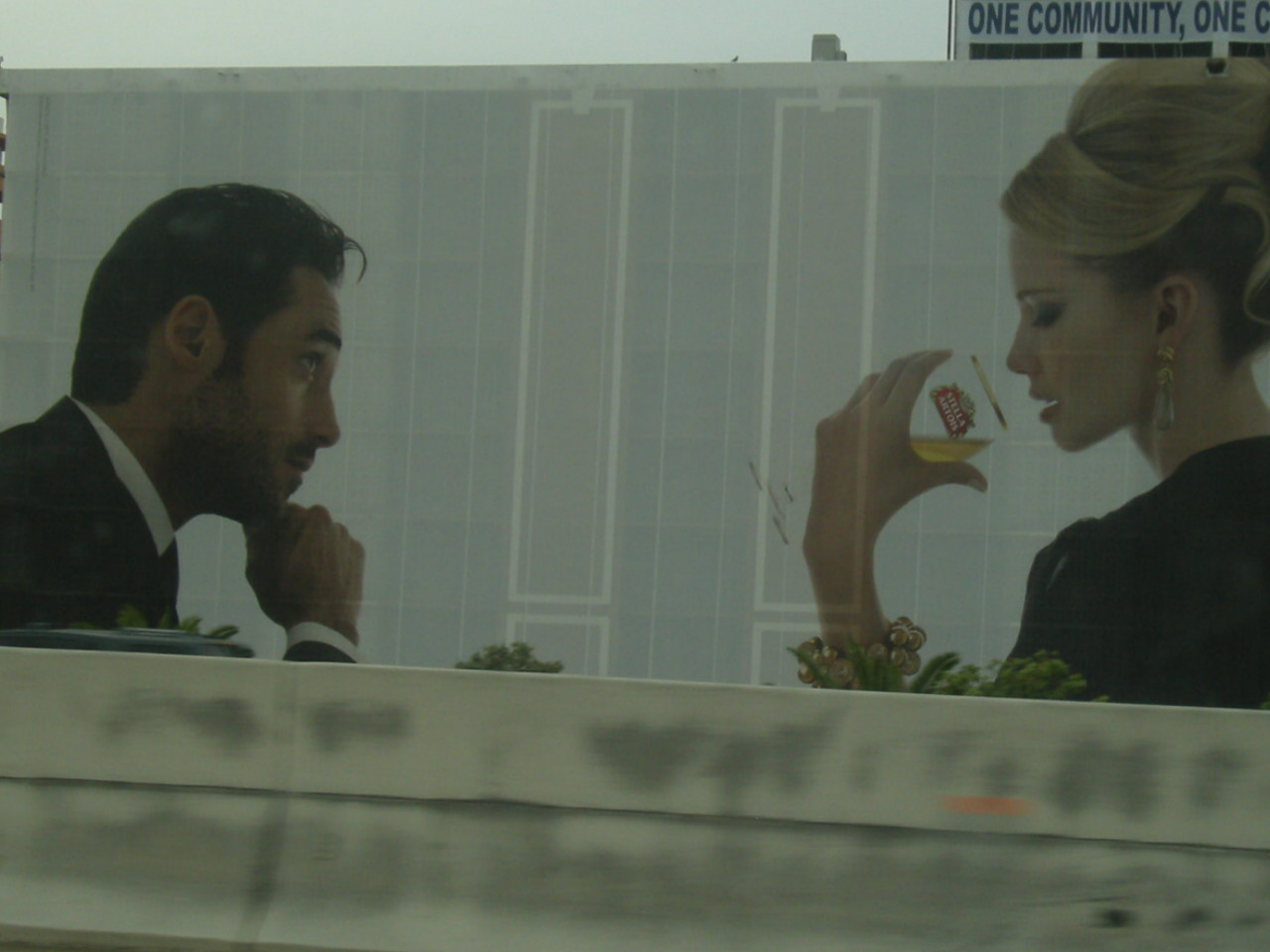This striking advertisement for Stella Artois beer is displayed on a large billboard or possibly a photorealistic mural painted on the side of a building. The upper three-quarters of the image are dominated by a scene featuring a man and a woman seated at a table. 

The elegantly dressed woman, with her blonde hair styled in a sophisticated beehive and wearing long gold earrings and a sleek black dress, is the focal point as she holds a champagne glass with the Stella Artois logo and a gold rim, just about to take a sip. Her gaze is entirely fixed on the glass, and the golden beer it contains, showing her appreciation and anticipation. 

Opposite her, the man, dressed in a black suit and white shirt with short dark hair and dark stubble, leans on his fist while looking at her intently, his curiosity piqued by her reaction. The setting, possibly a restaurant as suggested by the table adorned with flowers, creates an intimate and refined atmosphere. 

In the foreground, the concrete barrier of a road and a few potted plants are visible, with the sky and a building partially captured in the upper right corner, further grounding this sophisticated scene in an urban environment.